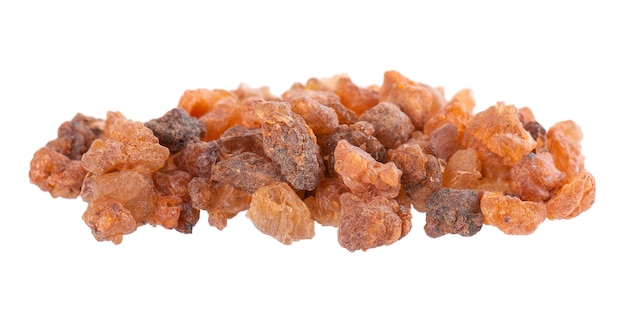The image displays a pile of small, irregularly-shaped rocks set against a stark white background. The rocks vary significantly in color, ranging from light orange and rust tones to dark brown, purple, and almost black hues. The pebbles, which are jagged and lack smooth edges, evoke an almost organic appearance, similar to dried fruit such as raisins or apricots. They form a clustered formation that might resemble a naturally occurring structure, like a finger-shaped rock formation. The detailed, close-up shot emphasizes the varied textures and colors of this intriguing mineral aggregate, suggesting it might be an illustration from an article about rocks or minerals.